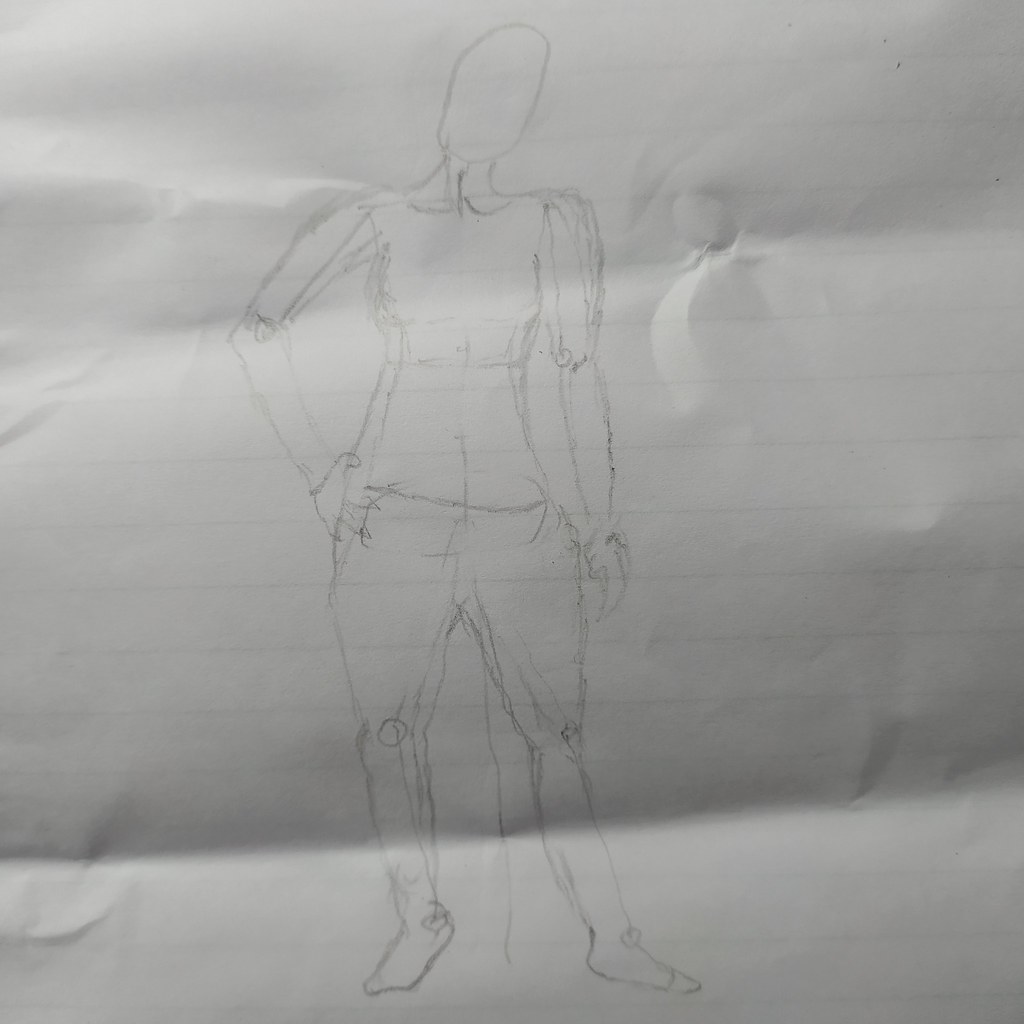The photograph depicts a pencil sketch drawn on crinkled, lined notebook paper. The sketch appears to be a rough study or practice drawing of a humanoid figure, reminiscent of a mannequin or crash test dummy. The figure lacks facial features entirely, presenting a blank, tilted head. Its body is composed of basic shapes connected at various joints, illustrated with noticeable circles at the ankles, knees, elbows, and hips, emphasizing posability. One hand rests on its hip while the other hangs straight down. The legs are drawn with thicker thighs, seemingly in accurate proportion to the rest of the body. The sketch, consisting solely of black and white pencil marks, is characterized by a rough, scribbled quality, suggesting the artist is learning or experimenting with drawing human anatomy.